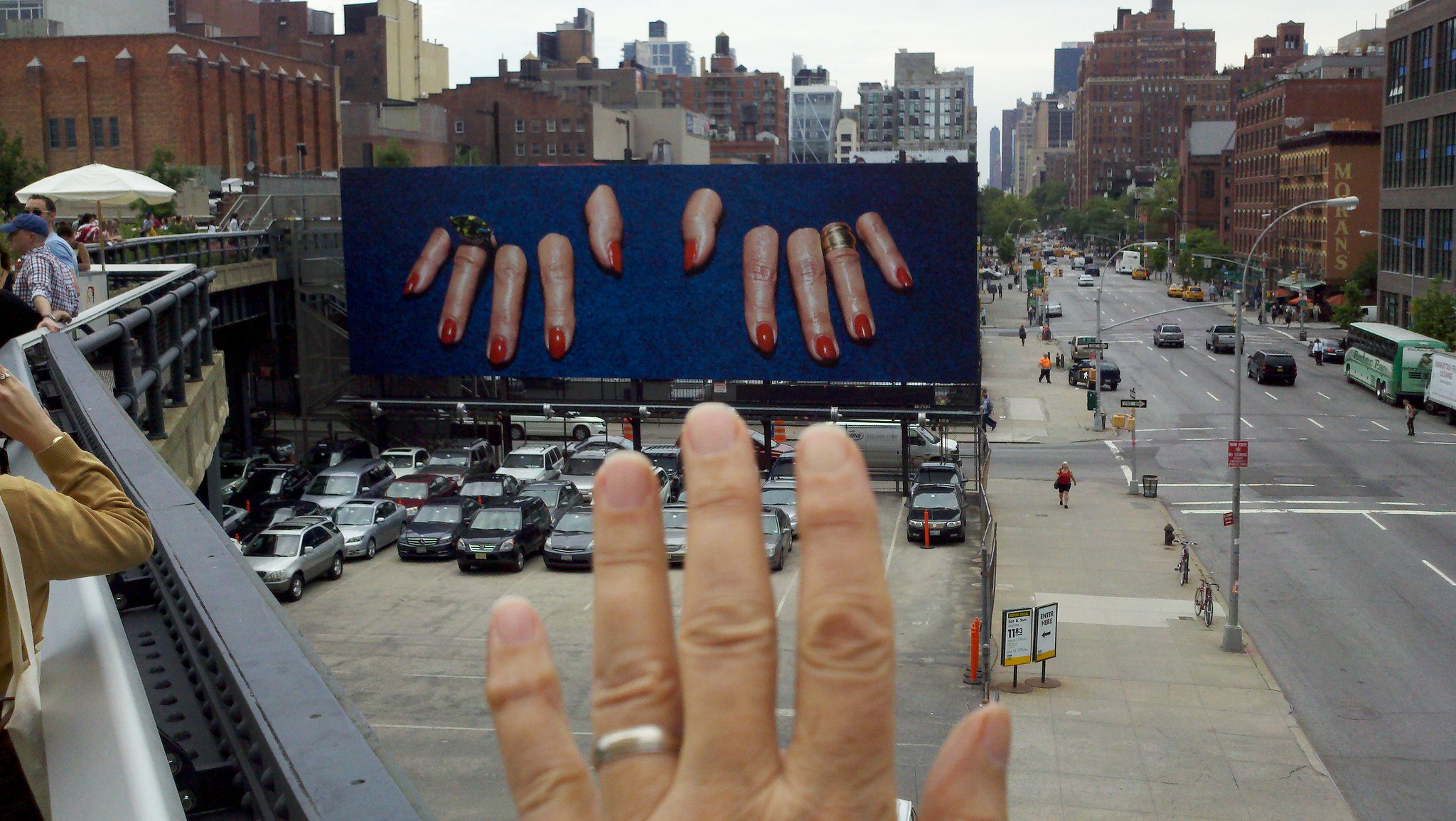In this photograph taken on an overcast day, the foreground features a white-skinned man's hand extending from the knuckles to the fingertips. He wears a wedding band on his ring finger, and he holds his hand up in front of the camera, aligning it with a distant billboard located at the edge of a parking lot. The elevated perspective reveals that the man is standing on a higher level while the billboard stands on a black metal scaffold. The billboard itself is royal blue, and intriguingly, two hands with red-painted fingernails protrude from behind the fabric, as though a woman is reaching through it. The man appears to be playfully positioning his fingers to interact with the billboard's hands. Below him, the parking lot is filled with numerous parked cars, and a busy four-lane urban road stretches out, surrounded by many tall buildings.